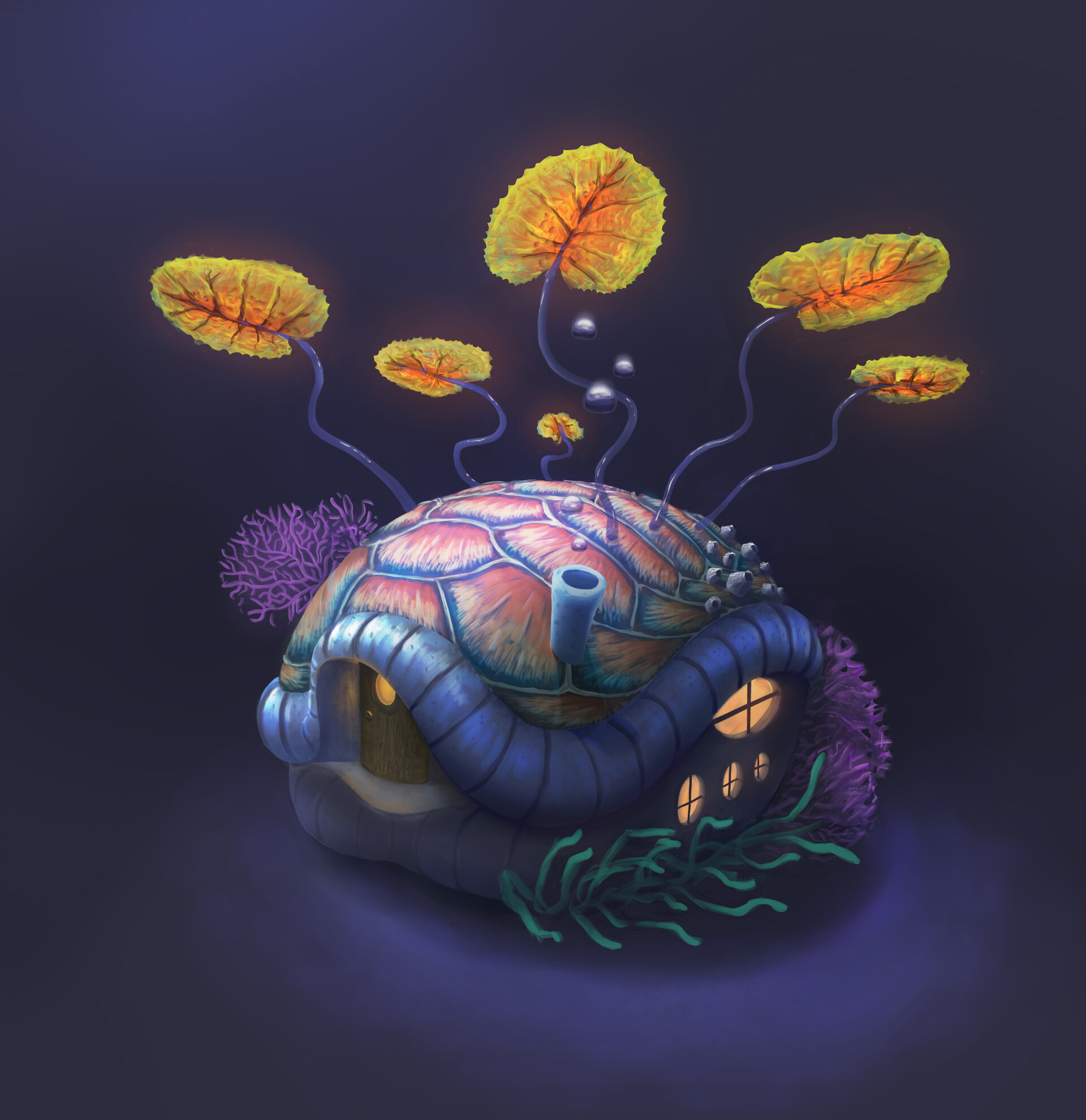The illustration is a digitally rendered, AI-generated drawing of a house ingeniously designed to resemble a turtle shell. The body of the turtle is absent, but where the turtle's head would be, there is a small wooden door with a knob and a tiny window. The shell's sides feature oval-shaped windows with frames, emitting a warm yellowish light that suggests the house is inhabited. The shell roof is adorned with a vivid color scheme of red, yellow, and green, creating a distinctive pattern. Emerging from the top of this shell are translucent blue and purple stems, curving gracefully and adorned with large, oval yellow leaves veined with orange. Additional greenery and seaweed—both green and purple—are seen at the base and sides of the house. A small blue chimney tops this imaginative structure, all set against a dark purple-black backdrop, hinting at an underwater or fantasy environment. The overall effect is a whimsical, detailed fusion of marine life and architectural creativity.